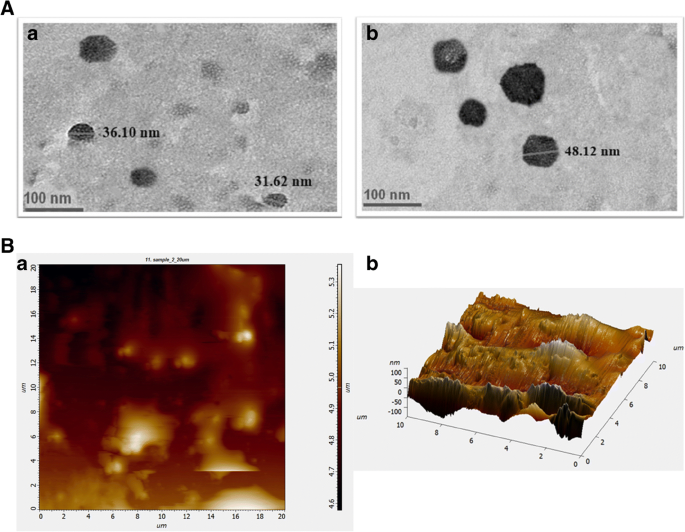The image consists of a composite of four individual pictures arranged in a square grid, labeled A and B for two distinct sections. The top half (Section A) features black and white microscope images showing close-up views of material with clusters of small black dots on a gray background. Specific measurements are indicated, including 48.12 nm, 36.10 nm, and 31.62 nm. The bottom half (Section B) contains two different types of visual data. In the lower left (image A), there is a detailed computer-generated elevation map, rendered in shades of brown and yellow, possibly representing topographical data or sensor readings, annotated with numbers and a color key. The lower right (image B) shows an axonometric projection with various numerical labels and color gradients, corresponding to micrometer and nanometer scales. This intricate compilation of visual data suggests a detailed scientific analysis of microscopic structures and their associated measurements.